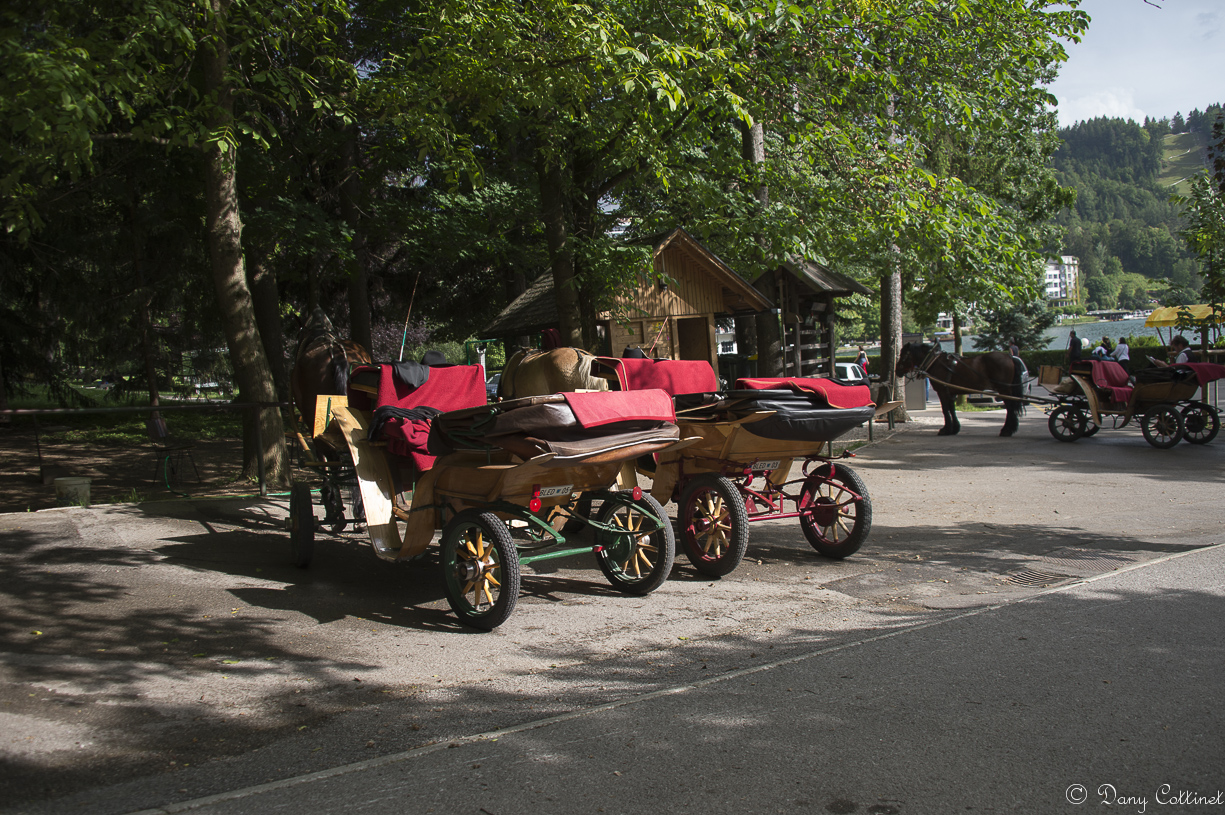The photograph captures a rustic outdoor scene featuring multiple horse-drawn buggies in what appears to be a camp or recreational area. Dominating the foreground are three open-topped carriages, two of which are painted red. The first carriage is pulled by a black horse, while the second, positioned to the right, is hitched to a tan horse. In the background, a third brown horse stands tethered near a yellow buggy with red seats. People can be seen both on the carriages and walking around, adding life to the setting. 

The left side of the image is framed by numerous trees with visible brown trunks and lush green foliage. Further back, almost center-right, there is a brown log cabin surrounded by additional trees and a sloped hill adorned with evergreen pine trees. The sky above is a soft whitish blue, lending a serene atmosphere to the scene. The street beneath the carriages and horses is composed of grayish concrete, contrasting with the natural surroundings. On the lower right corner of the photo, the watermark and name "Danny Corwin" are visible in white font. Lastly, towards the far end of the image, there appears to be a small lake and a business-like shed, nestled in what seems to be a valley framed by distant mountains.